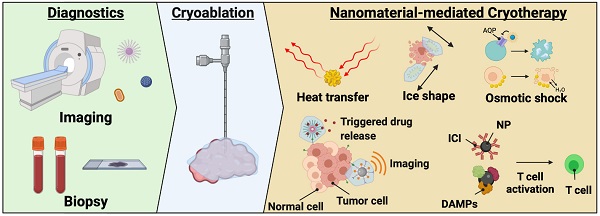This detailed and comprehensive illustration is a narrow, horizontal, rectangular graphic focused on cancer treatment procedures. On the far left, it features a green rectangle with an arrow pointing forward, labelled "Diagnostics," including elements like a CT scan machine, vials of blood, and a glass slide for cell examination under a microscope, captioned "Imaging" and "Biopsy." Adjacent to this is a white arrow marked "Cryoablation," represented by an image of a brain with a metal probe inserted into it. The largest section on the right is entitled "Nanomaterial Mediated Cryotherapy" and is filled with numerous images and technical terms that outline the steps involved in killing cancer cells. This section includes detailed references to "heat transfer," "ice shape," "osmotic shock," "triggered drug release," and "imaging," along with terms like "normal cell," "tumor cell," "DAMPs," "ICI," "NP," "T-cell activation," and "T-cell." The graphic as a whole serves as a visual guide to the stages and technologies used in advanced cancer diagnostics and treatment.